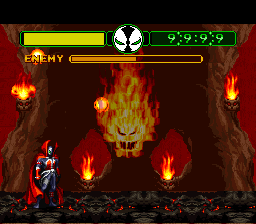Screenshot of a 2D fighting game. On the left side of the screen, a character stands poised for battle, facing off against an opposing character on the right. Both characters are set against a detailed backdrop, ready to fight each other. At the top left, a yellow health bar extends from the center of the screen to the left edge, indicating the player's health status. Approximately 10% of this bar is missing, suggesting the left-side character has already taken some damage. The score for the right-side character is displayed prominently in a numeric format at the top right corner, showcasing their progress in the game. The entire scene is vividly rendered, capturing the intensity and excitement typical of classic 2D fighting games.